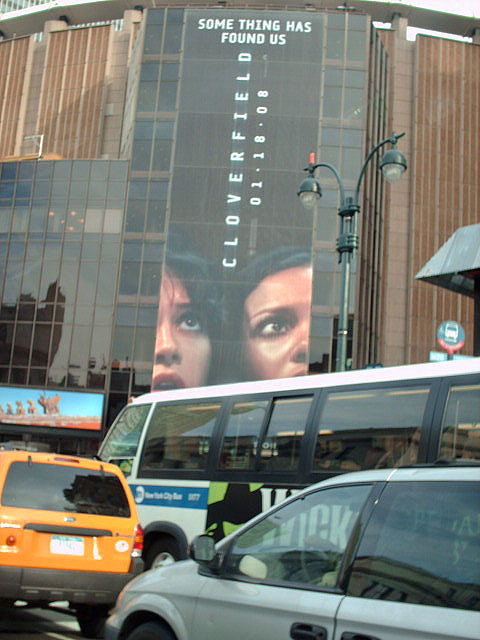In the foreground of the image, there is an orange vehicle with a flat back design. Just behind it, a portion of a gray station wagon is visible. Behind these vehicles, a white city bus is seen with black-framed windows and a distinctive blue stripe. Prominently displayed on the bus is an advertisement for the musical "Wicked," featuring a green background and the iconic image of the black-clad Elphaba, accompanied by the word "Wicked" in bold, white capital letters.

Beyond the vehicles, a tall building rises, appearing to be around six or seven stories high. The architecture of the building resembles an octagon but with many more facets, creating a shape that is nearly circular yet still angular with approximately twenty sides. Dominating the side of this building is a large advertisement with a black background, promoting the movie "Cloverfield." It features an ominous tagline, "Something has found us," along with an image of two women looking terrified and staring into the distance.